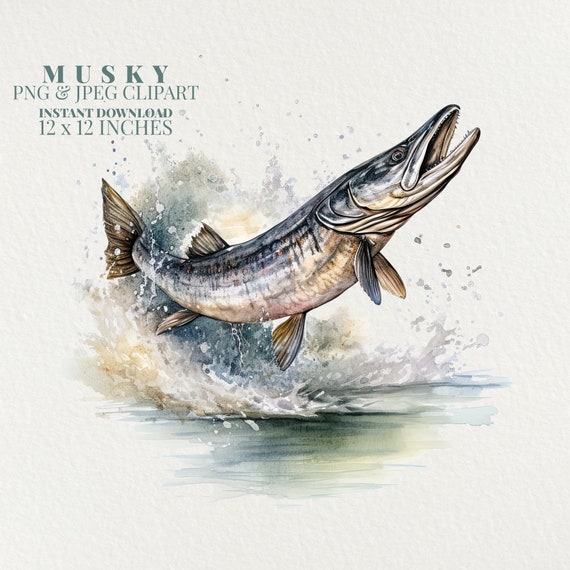The image depicts a detailed painting of a muskellunge, also known as a muskie, leaping out of the water. The fish appears large and is positioned with an arched body mid-leap, its mouth wide open revealing its teeth. The coloration of the muskie features a gray top, a greenish eye, and a beige-like color underneath the mouth, with variations of creams, tans, and dark grays throughout its body. Its fins and tail are also shaded in gray and tan. The water around the muskie is actively splashing and cresting, rendered in muted hues of gray, green, blue, and silver, mirroring the earth tones of the fish. The background has a poster-like quality with subtle details that include splashing water and the fish's reflection. The image is advertised as "muskie PNG and JPEG clip art" available for instant download in a 12 by 12-inch format.